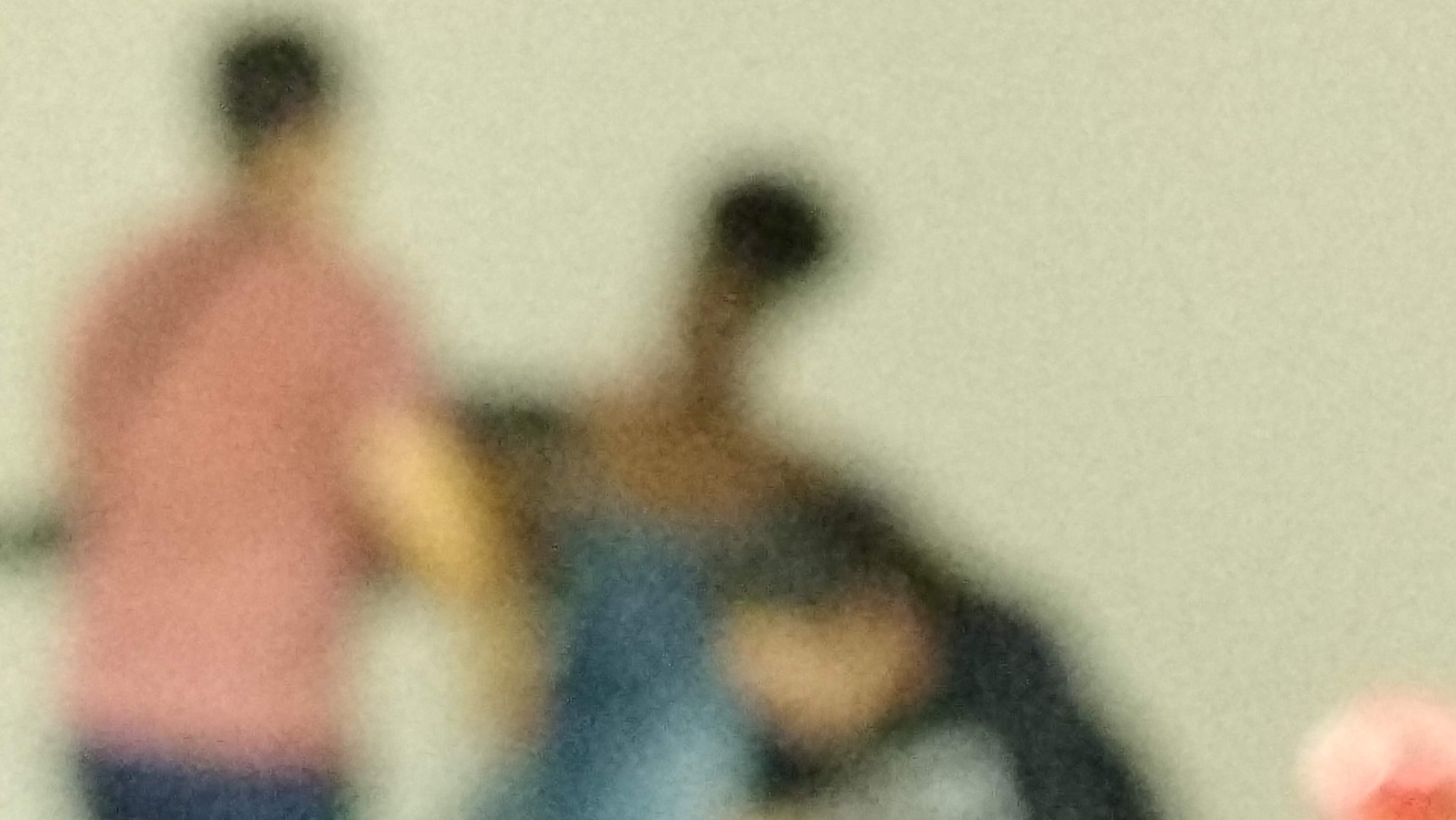The image depicts a heavily blurry scene where two individuals are seen dancing, though discerning precise details is challenging. The background is predominantly gray, while the bottom right-hand corner features the outline of a pink, spherical object. Its nature is ambiguous; it could be a flower or perhaps part of a banister, with a rose hue transitioning to a darker pink on the underside.

On the left side of the image stands a man dressed in a pink shirt and blue pants. He has dark hair and his arms are slightly outstretched towards his dance partner. To the right, facing the man, is a woman with a short afro hairstyle. She has darker skin and is wearing a blue dress that reveals a considerable portion of her shoulders. Additionally, she appears to be adorned in a flowing cape—either black or blue—that trails behind her, accentuating the motion of her dance.